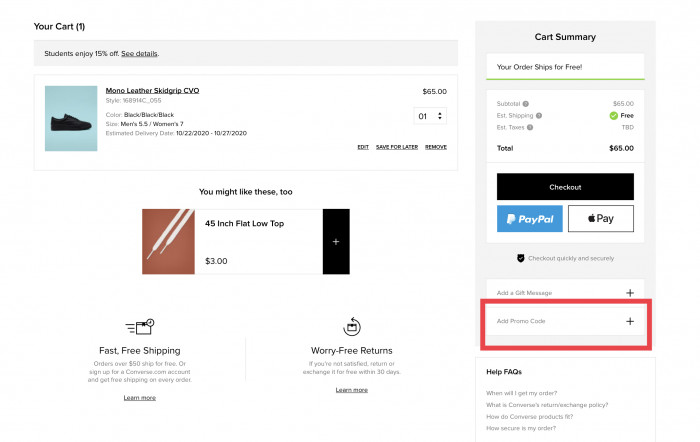This detailed caption describes a screenshot of an e-commerce purchase page. On the page, there is a section labeled "Your Cart," which shows one item added: a pair of shoes identified as "Monoletter Skid Grip CDO." The item specifics include style number 168914_055, color black, size men's 5.5 or women's 7. The price of the shoes is listed as $65, with free estimated shipping. The estimated delivery window is between October 22, 2022, and October 27, 2022. Below the cart summary, there's a suggestion for another product, a 45-inch flat low top shoes priced at $3. Additionally, there's a mention of "worry-free returns guarantee" and a section on the right with frequently asked questions for customer assistance. The total amount to be paid is $65.